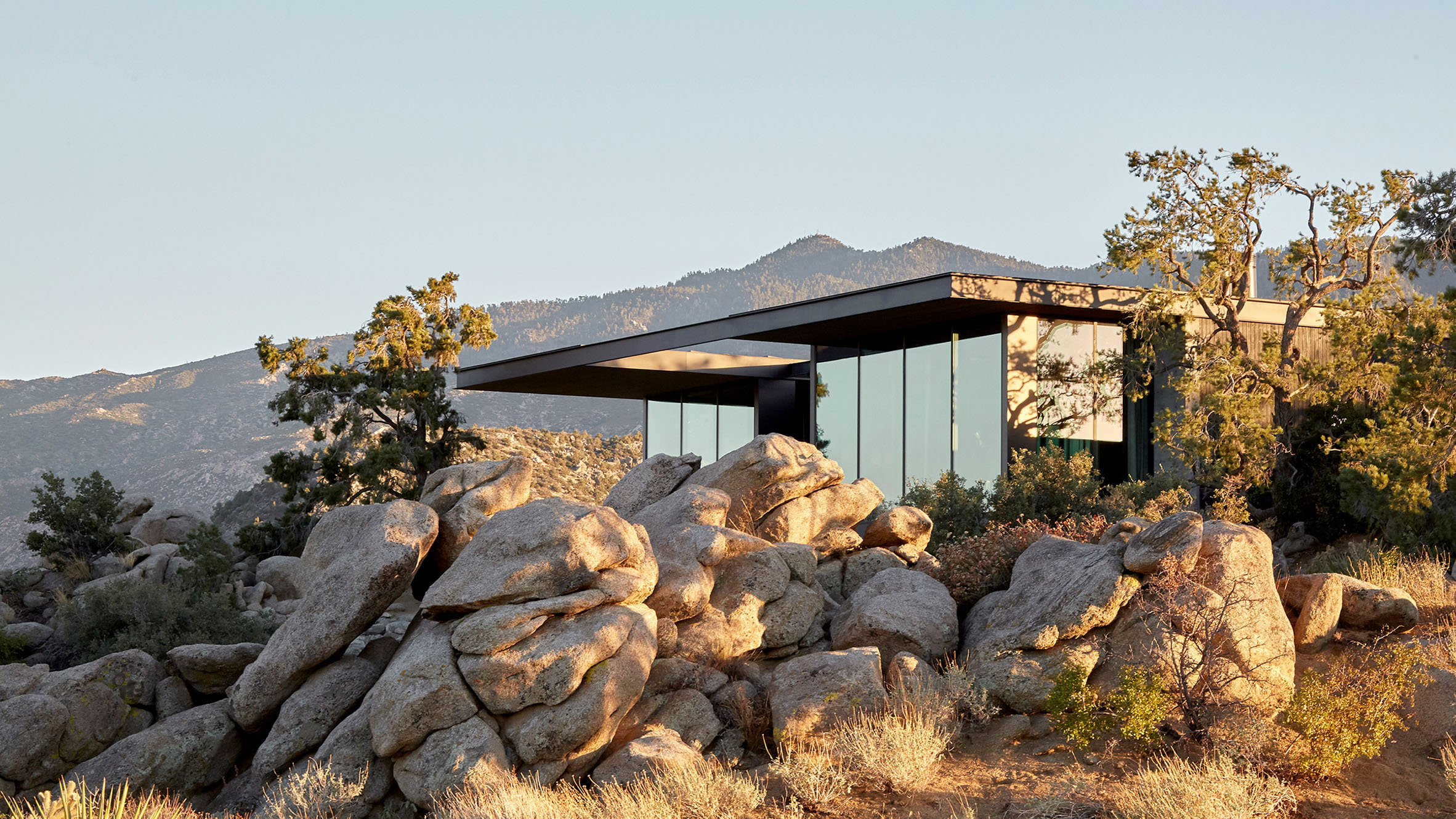The photograph showcases a modern, single-story house with a flat roof, prominently featuring floor-to-ceiling glass walls on its front side. It is set amidst a natural wilderness with no other man-made structures in sight. The foreground is characterized by light brown, irregularly shaped rocks and scattered bushes that appear dry and brown. Surrounding the house are wiry trees with thin green leaves and patches of green and brown grass. The house is situated on a hill, offering a striking view of a distant dark brown mountain. Meanwhile, the sky above is a muted light blue, adding a subdued, tranquil atmosphere to the scene.